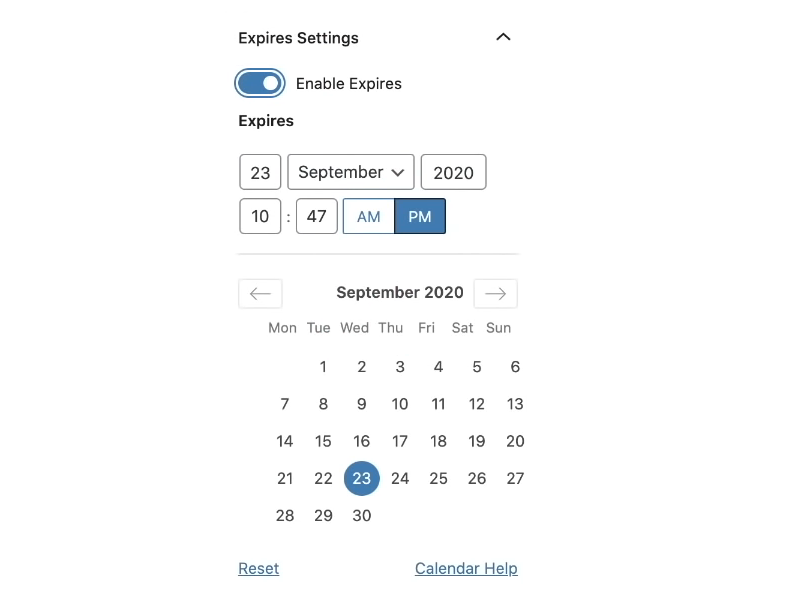The item depicted is a digital screen displaying a calendar and its settings interface for September 2020. The background of the screen is white. At the top left corner, in black letters, it reads "Expire Settings," accompanied by an upward caret symbol to the right. Below this line, there is a blue toggle button in the "on" position, with the label "Enable Expires" in black letters beside it. 

Further down, the heading "Expires" is displayed in bold black letters, followed by fields to set the date and time. The current setting is "23 September 2020, 10:47 PM." 

The calendar for September 2020 is centered on the screen, with the month and year labeled in dark bold letters at the top. Navigation arrows flank this label: a left arrow on the left side and a right arrow on the right side. 

The days of the week are listed on the next line in a horizontal row, ranging from Monday to Sunday. The month calendar shows that September 1st falls on a Tuesday and September 30th on a Wednesday, with each date indicated in black letters on a white background. 

The date "Wednesday, September 23rd" is highlighted with a blue circle, and the number 23 is displayed in white, indicating it has been selected. 

At the bottom of the screen, two options are presented: "Reset" on the left in blue letters, and "Calendar Help" on the right, also in blue letters. Both options are underlined, indicating they are clickable links or buttons.